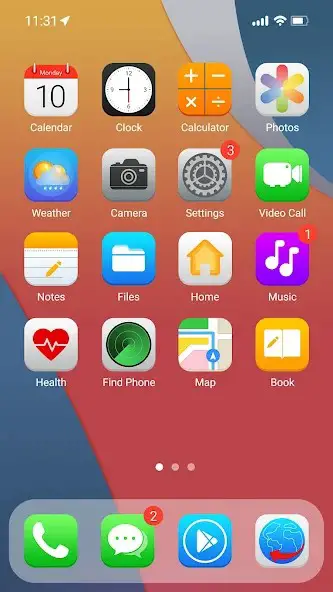This screenshot displays the home screen of a smartphone organized into a structured grid of app icons, each accompanied by their respective names. The icons are organized in five rows with four apps per row, followed by a row of four nameless app icons at the bottom. 

Here are the app icons from top to bottom, left to right:

1. Row 1: Calendar, Clock, Calculator, Photos
2. Row 2: Weather, Camera, Settings, Video Call
3. Row 3: Notes, Files, Home, Music
4. Row 4: Health, Find Phone, Map, Book

The bottom row consists of four icons without text labels representing:
1. A green phone call app
2. A green messaging app
3. A blue video player app
4. A blue globe with a white background, possibly a web browser

The background showcases an abstract design featuring a diagonal, curvaceous orange gradient line intersected by darker blue lines, adding a vibrant and modern touch to the home screen.